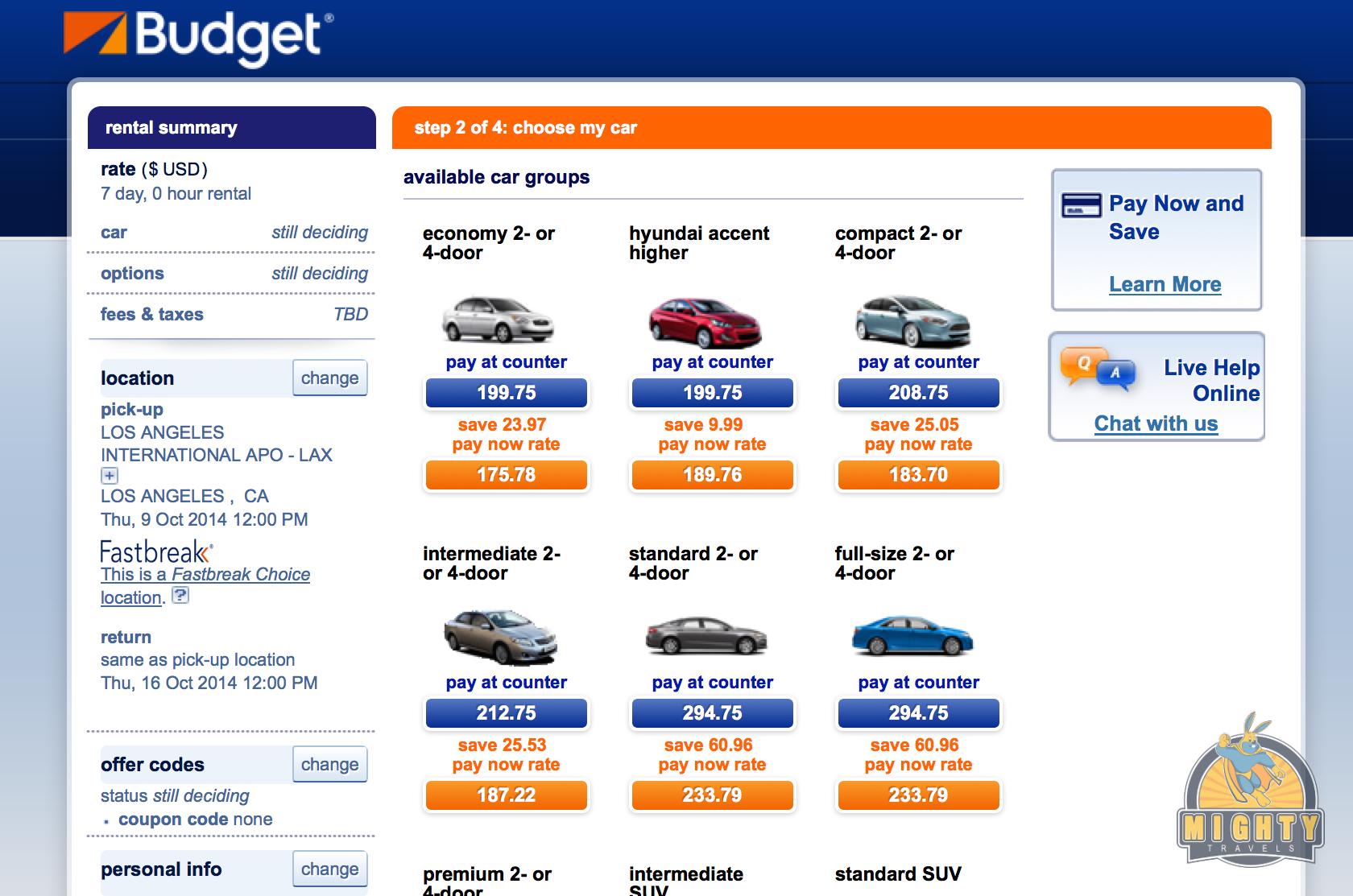Screenshot of a car sales website named "Budget," showcasing six different cars available for purchase. Located at the top left corner is the website's name. In the center of the image, each car listing is displayed with detailed information:

1. The first car is labeled as "Economy," featuring options for either 2 or 4 doors. The displayed image shows a silver car. The listed prices are $199.75 if paid at the counter and $175.78 if paid online.
2. The next listing showcases a Hyundai Accent, highlighted in red. This compact car is also available with 2 or 4 doors, priced at $189.76.
3. The third car is categorized as "Compact" with options for 2 or 4 doors, priced at $183.70.
4. The fourth car is labeled "Intermediate," accommodating options for 2 or 4 doors, with a price tag of $187.22.
5. The fifth car is categorized as “Standard,” also with 2 or 4 door options, priced at $233.79.
6. The final listing is for a "Full Size" car, available with 2 or 4 doors, and is also priced at $233.79.

The image provides a clear and structured view of various car options, prices, and configurations available on the Budget car sales website.